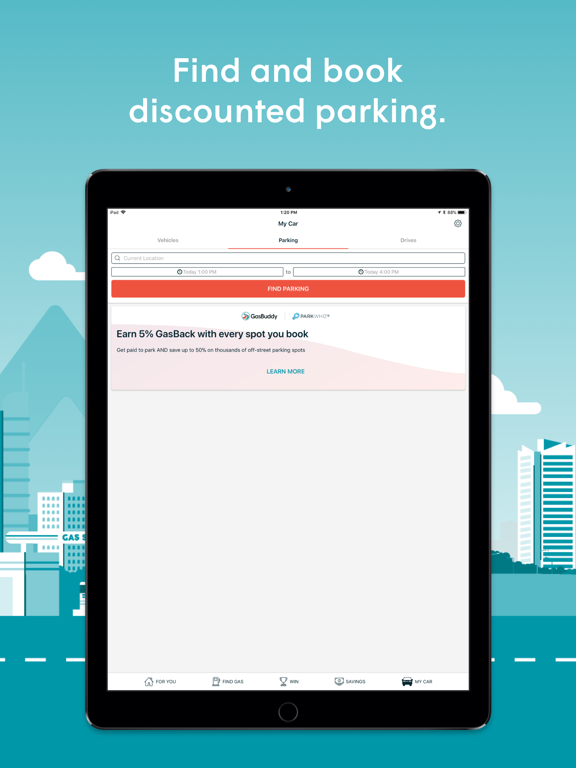The image is a screenshot of a vibrant advertisement featuring a black tablet against a predominantly aqua-colored background. The center of the image, which occupies about three-fifths to two-thirds of the screen, showcases the tablet with a lit white screen. 

In the background, text reads in white lettering: "Find & Book Discounted Parking." Accompanying this text is an illustrated scene featuring mountains, several clouds, various buildings, a "Gas" sign, and a road with white dotted lines. This backdrop sets an urban, travel-related context.

Prominently displayed at the forefront is the tablet interface, labeled at the top with "My Car," along with battery life and other standard tablet indicators. The interface lists three categories: "Vehicles," "Parking" (which is highlighted in black with a red underline), and "Drivers." Below these categories, there is a search function where users can enter a location, select a start time (shown as "Today 1 p.m."), and an end time (shown as "Today 4 p.m.") to find parking options.

At the bottom of the ad, white text on the tablet screen reads: "GasBuddy - Earn 5% GasBack with every spot you book. Learn more." This text promotes an incentive for booking parking through the app, reinforcing the benefits of using the service.